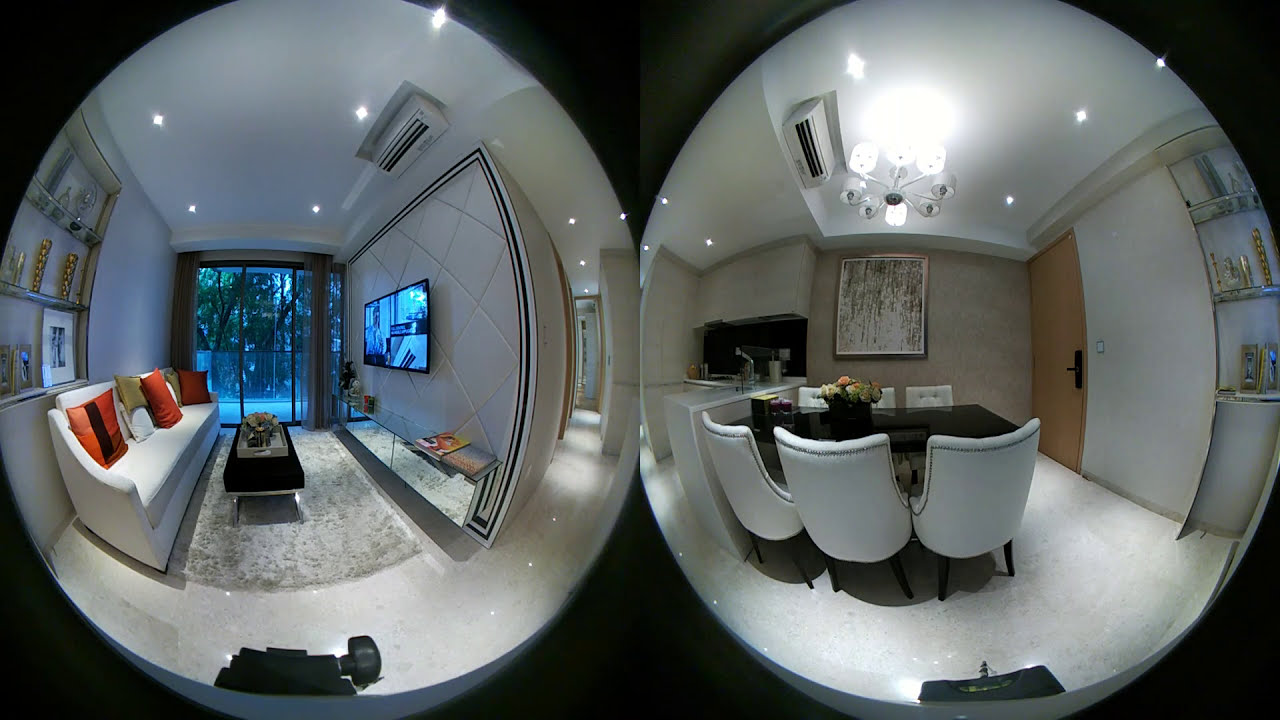The photograph depicts two fisheye lens, dome-like spherical views of different areas within a designer house, accentuated with a virtual reality panoramic effect against a black background. The left sphere showcases a plush living room, featuring a white sofa adorned with three red pillows and one gold pillow. A black coffee table occupies the space in front of the sofa, strewn with small objects, leading up to a wall-mounted flat-screen TV with a table beneath it displaying some magazines. Behind the couch, various decorative photos and objects adorn the wall, and a floor-to-ceiling sliding glass door reveals a view to the outside. The right sphere offers a glimpse into a sophisticated dining area, where a black rectangular table is surrounded by six white, puffy chairs. Above the table hangs a striking white chandelier, which adds to the room's elegant ambiance. The background reveals further details, including a stove and a brown wooden door, complemented by paintings and a shelf mounted on the walls. The cohesive color scheme of white walls ties both scenes together, suggesting they might represent connected spaces within the same stylish home.